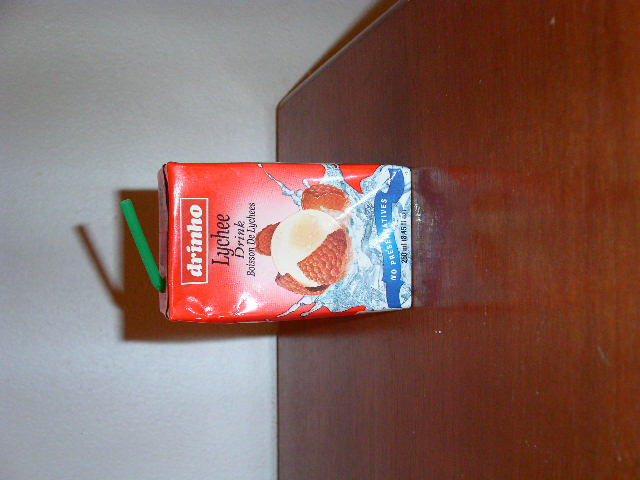The image showcases an indoor color photograph of a red rectangular juice box from the brand Drinho, featuring a lychee-flavored drink. The photo has been tilted 90 degrees counterclockwise which results in the wooden table, with a dark maple or cherry hue, appearing along the right edge of the image with a shadow visible. The backdrop includes a white wall with a light reflection. The lychee drink box, positioned on the table, has a green straw poking diagonally upwards from the top left, revealing a predominantly red label. The front of the box displays an image of a white lychee fruit, partially surrounded by chocolate candies and water gushing out. The brand name "Drinho" is marked in a red rectangle at the top, with the word "Lychee" spelled vertically beneath it.